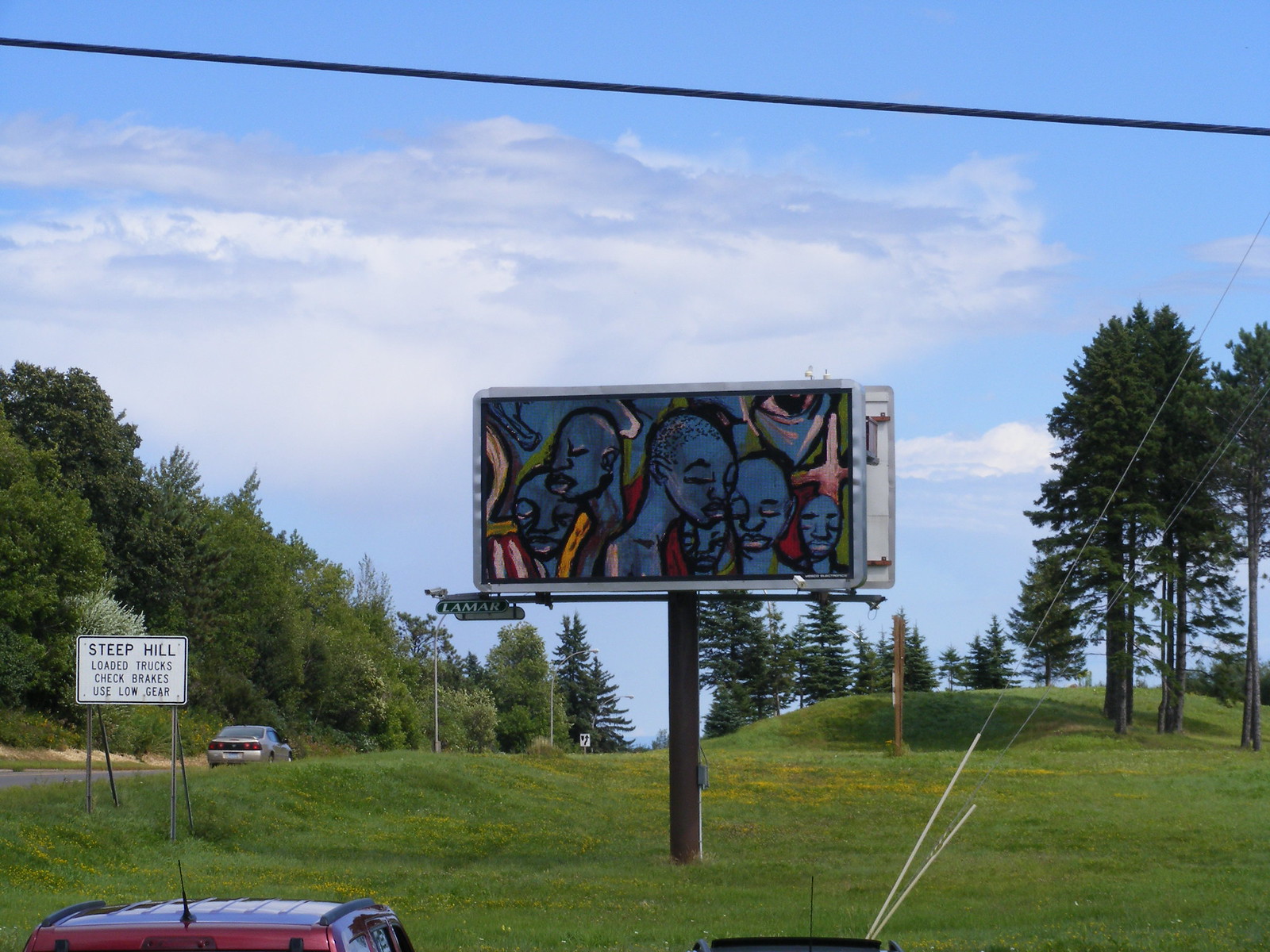A large billboard positioned at the edge of an intersection features an intricately painted mural, devoid of any commercial advertisements. The artwork, created with spray paint, vividly depicts six human figures, each seemingly engulfed in deep sorrow or mourning. The figures are characterized by a dark blue hue, adding to the somber atmosphere of the scene. Surrounding the mourning figures are detailed trees, which further enhance the emotional intensity and depth of the mural.